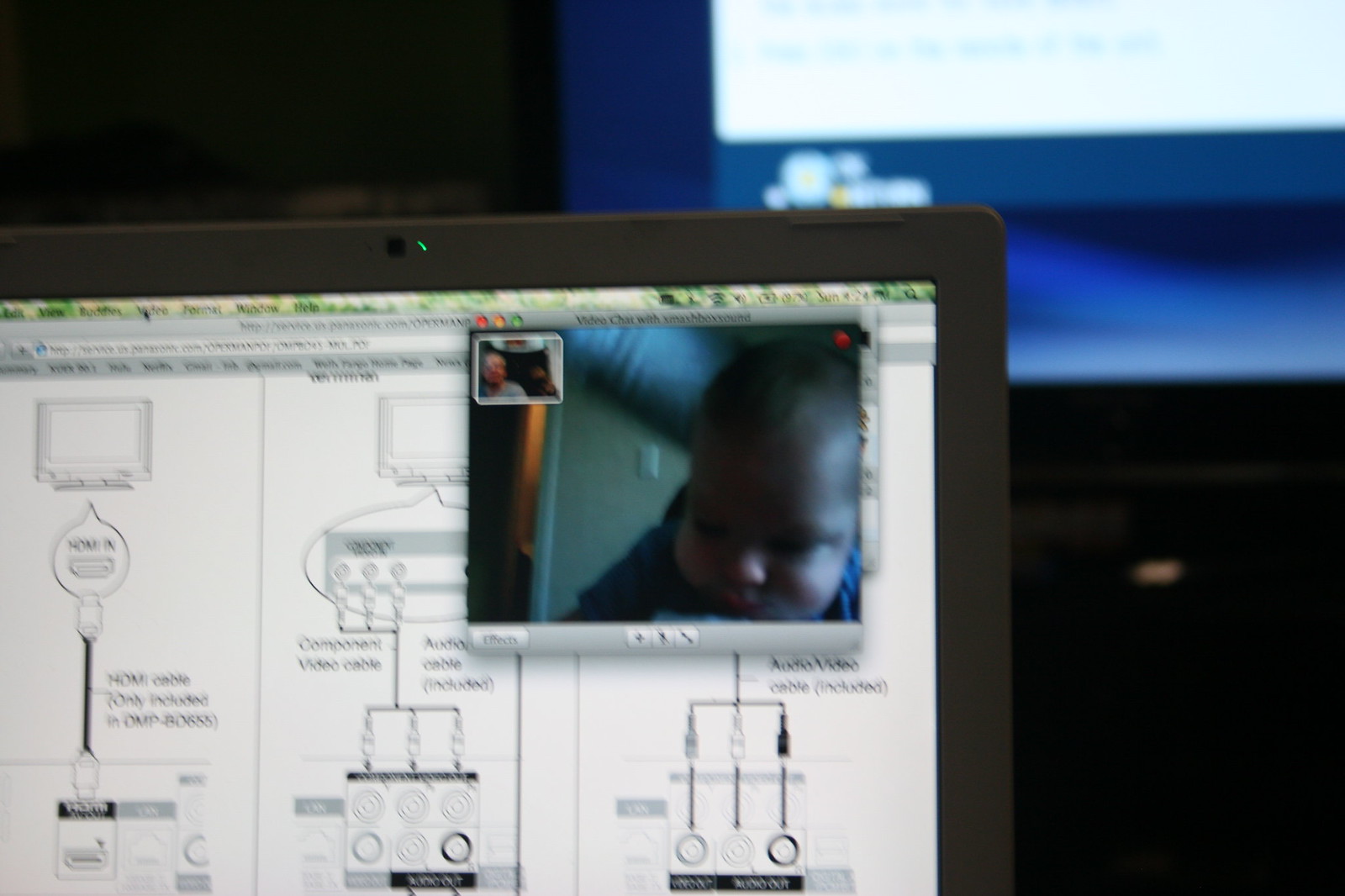The image depicts a close-up of a laptop screen, with a projector screen in the background. The laptop screen's frame is black with a small green light at the center top. On the laptop screen, a white background displays a detailed schematic showing how to connect various audio and video cables, such as HDMI, audio out, and audio in. In the upper right corner of this screen, there's a smaller video chat window showing a baby, likely monitored via a security cam. In the upper left corner of the same video chat window, there's a thumbnail of a man, possibly interacting with the baby. Behind the laptop, the projector screen shows an out-of-focus presentation with a blue background and scattered white rectangles, likely containing text. The surrounding area of the projector screen is mostly dark, creating a contrast that emphasizes the blue of the projected presentation.